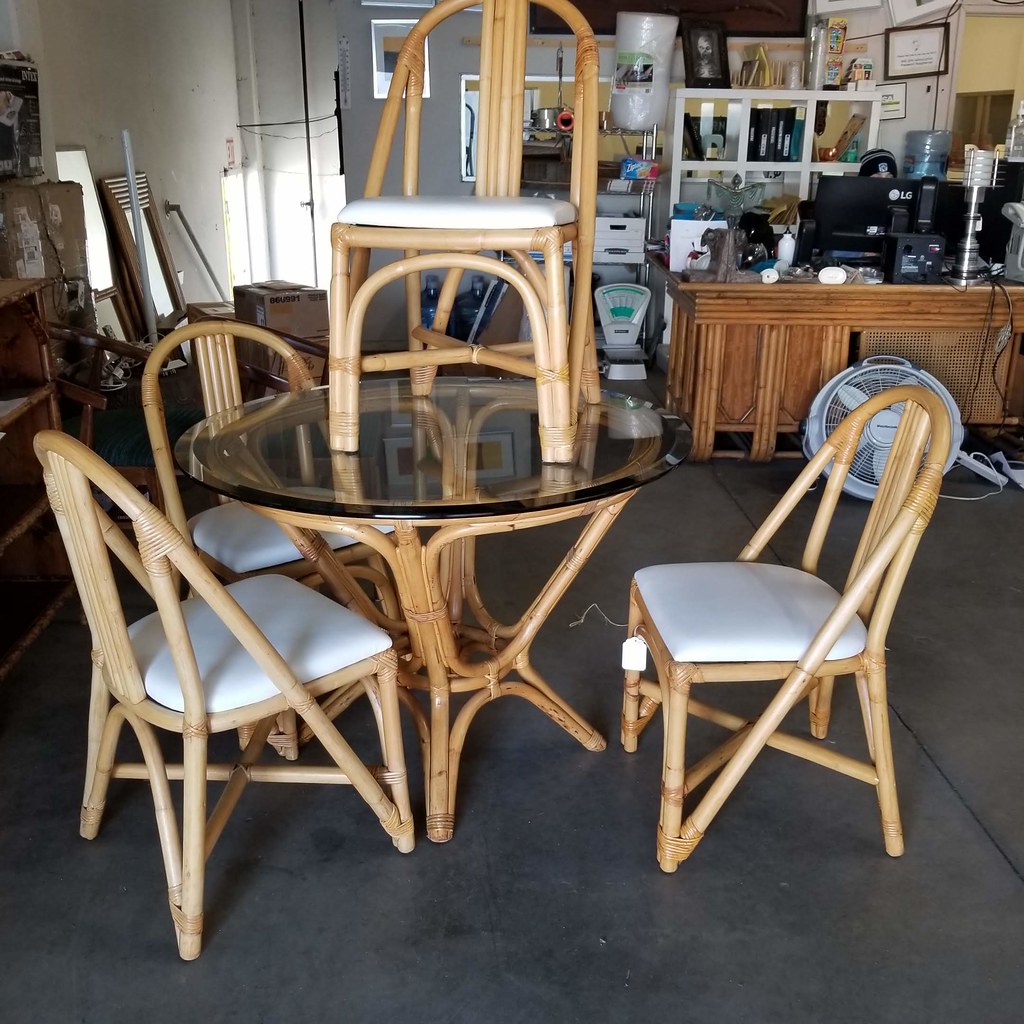The image depicts a somewhat cluttered room resembling a consignment or thrift store, filled with various objects all bearing price tags. Centered in the photograph is a round, smoked glass-top table supported by a light brown wicker or bamboo frame with four legs and intricate bindings. Surrounding the table are four terrace-style wooden chairs, also crafted from wicker material with rounded backs and white seat cushions; notably, one chair is perched atop the glass table. The floor beneath is gray, and to the left of the image, there's a bookshelf. On the right, a counter crowded with items borders the scene, with a white fan on a pole lying on the floor nearby. In the background, a messy bar area features a person sat behind an LG monitor, further suggesting that this setting is a store selling everyday items and furniture. Scattered around are additional items such as a lamp, a statue, an old-fashioned scale, and mirrors on the wall, contributing to the overall cluttered aesthetic.